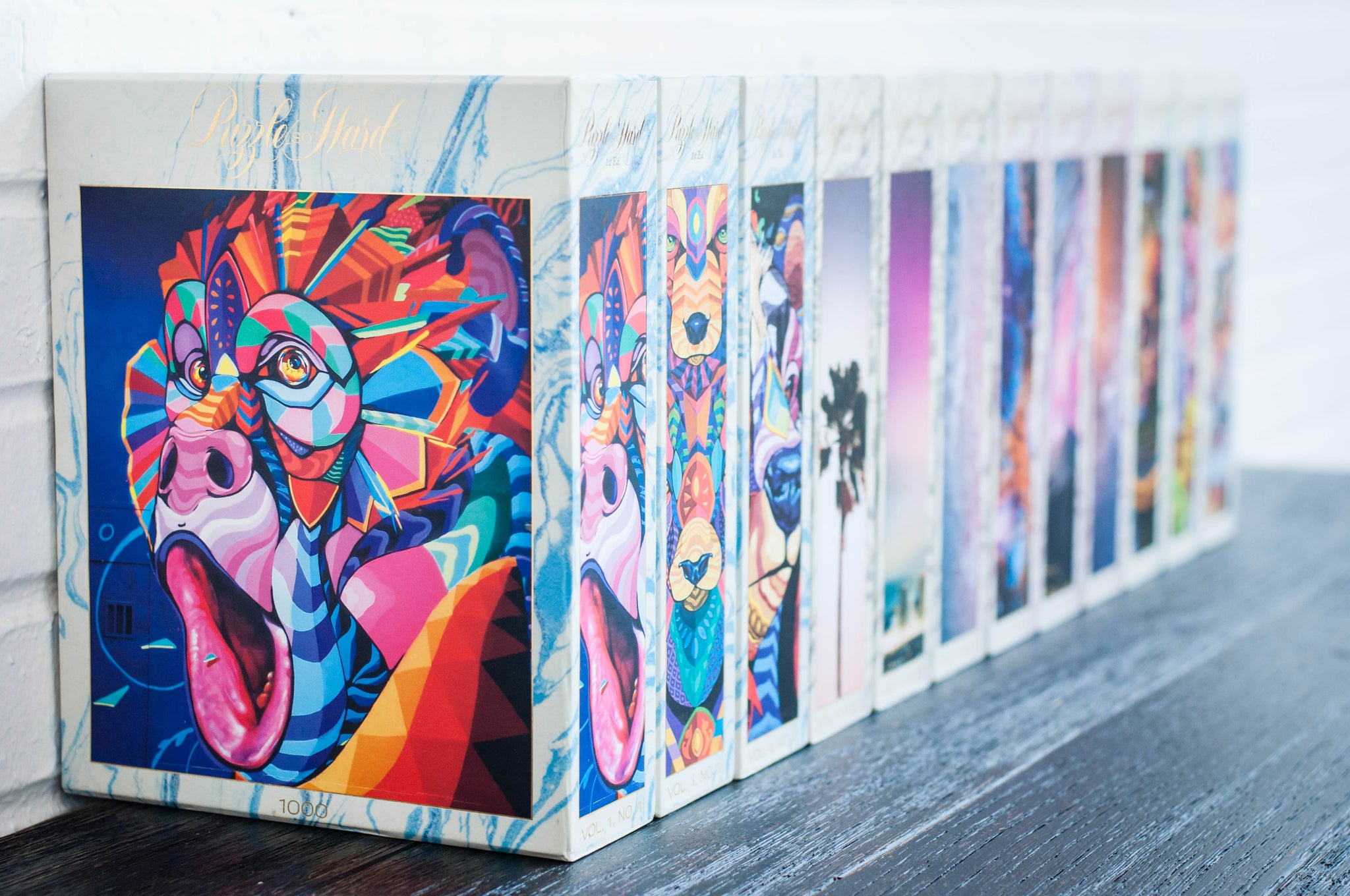This photograph captures a row of jigsaw puzzle boxes meticulously lined up on a dark brown wooden table. The boxes, which are uniform in shape and size, appear to be from the same company and feature a marbled white design with blue streaks. Against a backdrop of white painted brick, the boxes stretch into the distance, becoming gradually more blurred, with approximately ten boxes visible.

The front cover of the nearest box features a striking, brightly colored geometrical depiction of a howling monkey face, rendered in diverse shades such as light blue, teal, orange, yellow, and green. The monkey's eyes and mouth are depicted wide open in an abstract style. Each box spine showcases a sample of the puzzle image contained within, hinting at the colorful and abstract art themes found inside. The text on the box reads "Puzzle Hard" in elegant gold cursive writing, adding a touch of sophistication to the vibrant display.